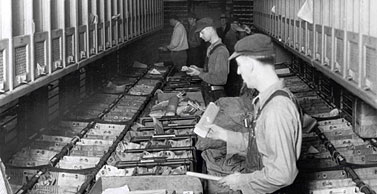This captivating 1950s black and white photograph depicts a narrow, rectangular room bustling with activity. The indoor scene, illuminated by artificial light, shows five workmen clad in long-sleeve coveralls and black caps meticulously sorting and classifying numerous boxes of mail. They appear to be in a mail office, with cabinets and drawers laden with copious amounts of mail. The men are each engrossed in their tasks, pulling items from the boxes in front of them and closely examining their contents, contributing to a sense of dedicated labor and organization. Despite the room's confined space, leaving little room to maneuver, it is lined with windows allowing an overseer to monitor the work being done. This image, devoid of visible ceiling or floor, captures a quintessential mid-century workplace brimming with mail and the diligent workers ensuring its proper handling.